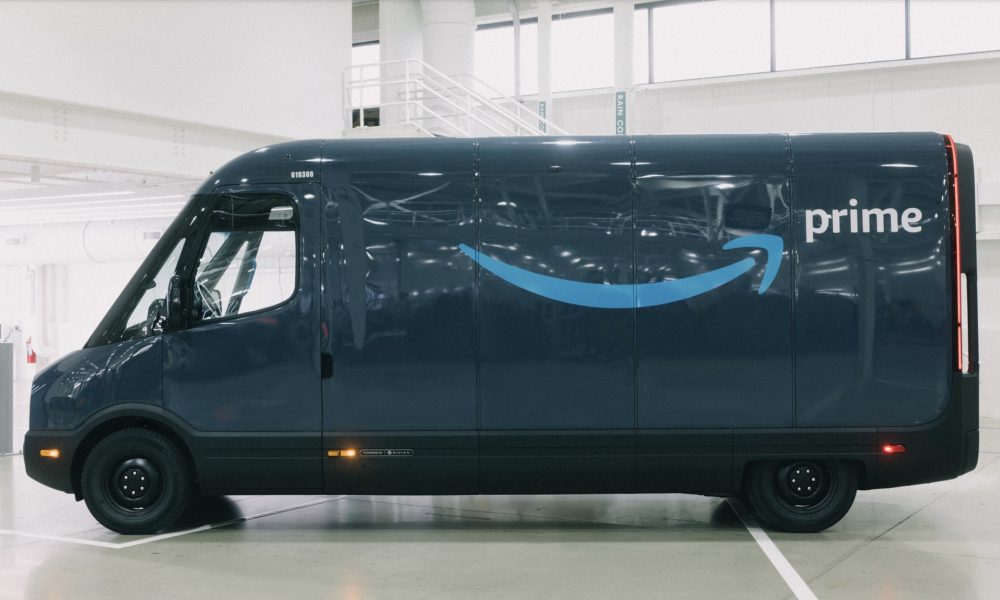The image features a seemingly new Amazon Prime delivery van positioned prominently in the center of a sterile, plain white room. The van appears to be a slightly longer, more modern model than the traditional Sprinter vans commonly seen on the roads. Its exterior sports a fresh sheen, indicative of a vehicle that has not yet been put into operational use. The setting suggests that this might be a factory or inspection area where the van is undergoing final reviews before deployment.

The environment surrounding the van is minimalist, accentuating its central position. The only other notable element is a red fire extinguisher placed far to the left, adding a splash of color to the otherwise monochromatic scene. The iconic word "PRIME" is prominently displayed on the back of the van, adhering to Amazon's usual branding. The van itself is finished in the typical Amazon blue, complete with the signature light blue swish logo. Overall, the image exudes a sense of newness and preparedness, poised right before the van embarks on its delivery journeys.